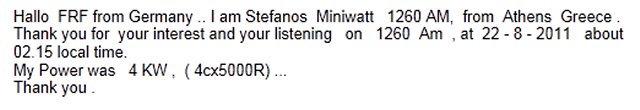The image depicts a screenshot of a text or email, formatted in a standard Arial font with black text on a white background. The message reads: "Hello, FRF from Germany, I am Stephanos Miniwatt, 1260 AM from Athens, Greece. Thank you for your interest and your listening on 1260 AM at 22-8-2011, about 02:15 local time. My power was 4 kilowatts (4CX5000R). Thank you." The text spans five lines with uneven spacing, where some words have unusually large spaces between them.